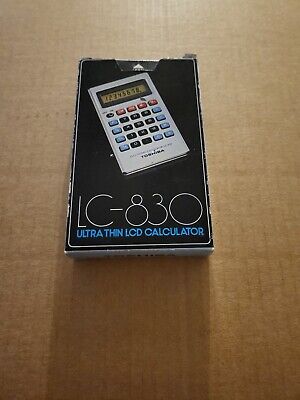This photograph captures a slightly worn, black rectangular cardboard box sitting on a brown piece of cardboard, with light casting a shadow toward the bottom. The box, which appears aged and has beaten-up edges, houses an analog-style calculator. The calculator is prominently displayed on the front, tilted slightly towards the top right corner. It has a white body with an LED screen displaying the sequence "1, 2, 3, 4, 5, 6, 7, 8". The buttons are a mixture of colors: the first and last rows are sky blue, the top row features smaller red buttons, and the remaining buttons are black. The white text at the bottom of the box reads "LC-830" and in blue text below, "Ultra Thin LCD Calculator". A small logo, likely Toshiba, is visible at the bottom of the calculator. The box has a thin white rectangular border and an arrow indicating where to lift to open the box. The overall color scheme of the image includes brown, black, white, light blue, and red.